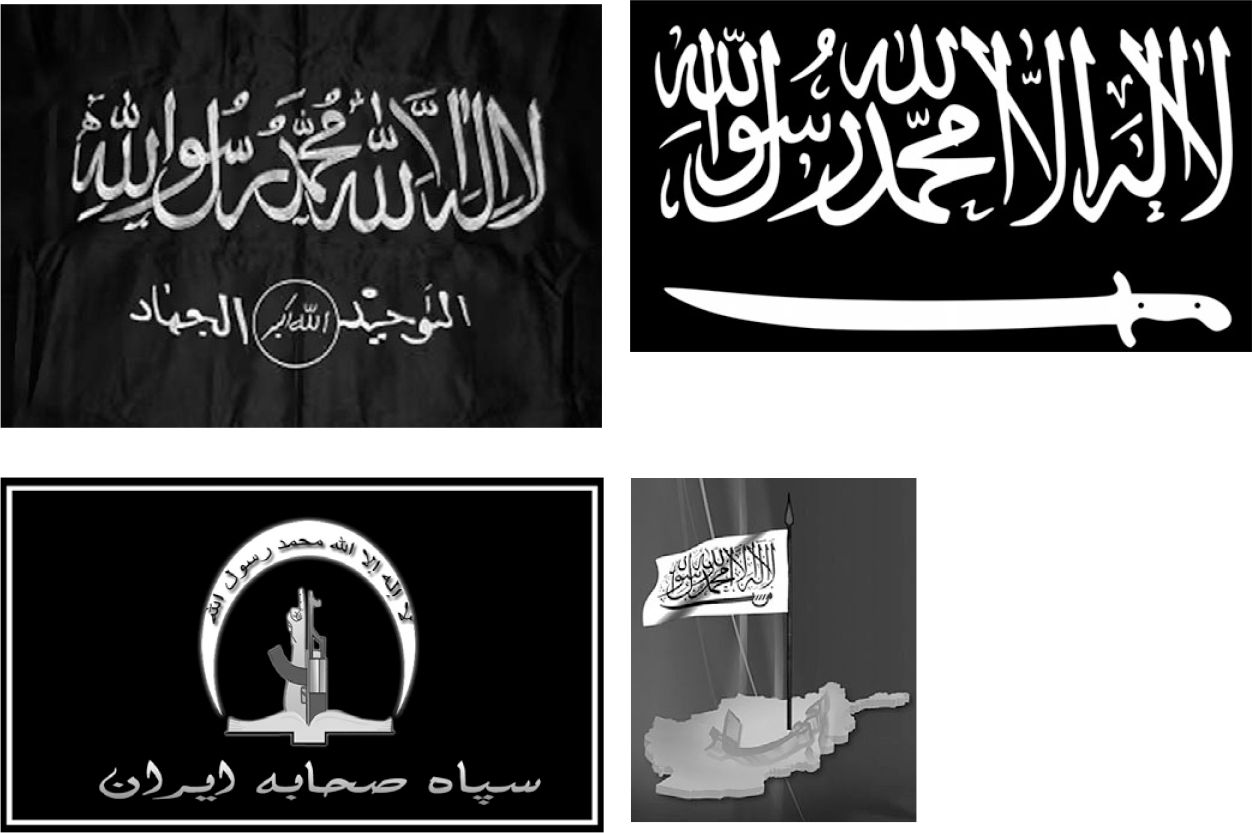The image is composed of four black and white panels arranged in a grid, three of which are horizontally oriented long rectangles in the top left, middle, and bottom left positions, with the fourth panel being a vertically oriented long rectangle in the bottom right. Each panel features white text on a black background, written in what appears to be Arabic or possibly Egyptian or another Asian language. 

The upper left panel resembles a piece of fabric, possibly a flag, with substantial Arabic text at the top and smaller writing at the bottom, centered within a circle that contains a small crown-like symbol. To its right, in the upper right, is a stark black panel with a large white sword lying horizontally at the bottom. The lower left panel showcases a book lying open, with an arm holding a machine gun placed over it and a crescent moon above the book, all superimposed with additional Arabic text. The bottom right panel portrays a black and white flag planted in the outline of a country, likely Afghanistan, suggesting a context tied to Islamic flags often associated with militant groups like ISIS. The overall tone of the images is stark, monochromatic, and includes elements symbolizing conflict and sovereignty.